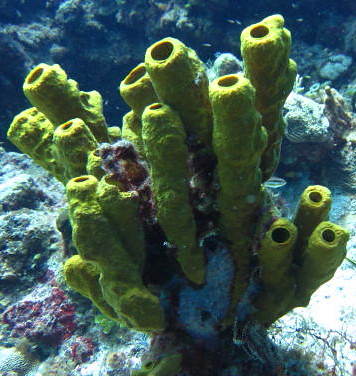The underwater photograph showcases a vibrant underwater scene dominated by a large, bright lime green coral in the foreground. This intricate coral features numerous tubular structures with circular tops, some exhibiting a distinct rust color in their interiors. Adjacent to the green coral on the left side, vibrant red coral and scattered rocks add to the scene's richness. The background reveals additional rocks and varied underwater vegetation lying on the ocean floor, all enveloped by the blue tinge of the water. To the right of the main coral, small fish can be glimpsed swimming near white, rough rocks, further enhancing the underwater tapestry.